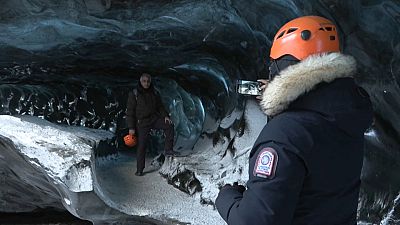In this photographic image set in an indoor or outdoor icy cavern, a man in a blue insulated winter jacket with a furry collar and an orange helmet stands with his back to the camera, capturing a photo using a phone. A patch, red and white but unreadable, is on his left shoulder. The setting is an ice cave, characterized by a white, likely snowy floor and a shiny, silvery rock on the bottom left corner. The dark ceiling above has hints of dark blue accents, and reflective surfaces line the wall. On the right side of the image, the man being photographed stands in focus, holding an orange helmet and wearing glasses, with white hair. He is dressed in black from his coat to his trousers, and one leg rests on a rock. To his right, there are several white structures or items, possibly covered in snow. This detailed scene captures the moment as he emerges from the icy cave, looking directly at the camera.